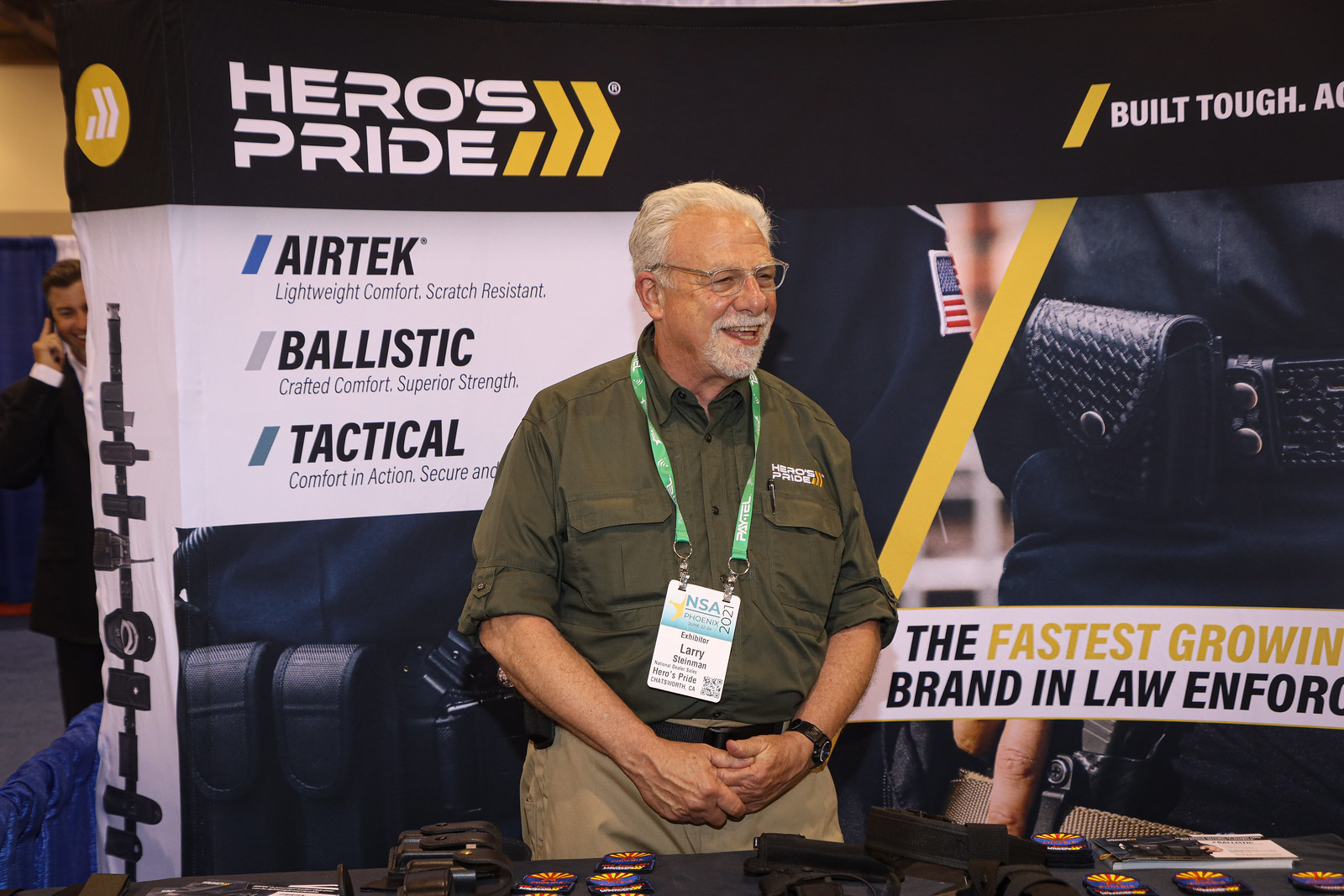This photograph features an older man, likely in his 60s, with short white hair, glasses, and a white goatee and mustache combination. He is dressed in an olive green short-sleeved button-down shirt that says "Hero's Pride" above one of the breast pockets, and he wears a lanyard around his neck, suggesting he is at a conference or trade show. His arms are crossed in front of him with his hands interlocked, and he is wearing a black belt and tan-colored pants, partially obscured by a table filled with various objects.

The background is filled with signage and promotional banners. Directly behind him is a banner with the Hero's Pride logo on a black background in white letters. Below that, there are words like "Airtek," "Lightweight Comfort," "Scratch Resistant," "Ballistic Crafted Comfort," "Superior Strength," "Tactical Comfort," and "Action Secure," although some of this text is obscured by the man. To his right, another banner proclaims, "The Fastest Growing Brand in Law Enforcement." Also visible on his right is an image of a police officer's belt with a clearly visible gun holster. The signs have a mix of white and black backgrounds with highlighted bullet points in blue and gray. The entire scene suggests a presentation or showcase for a law enforcement-supporting company, Hero's Pride, at a professional event. The man has a friendly demeanor and appears to be engaged with the audience or an individual off-camera to his right.